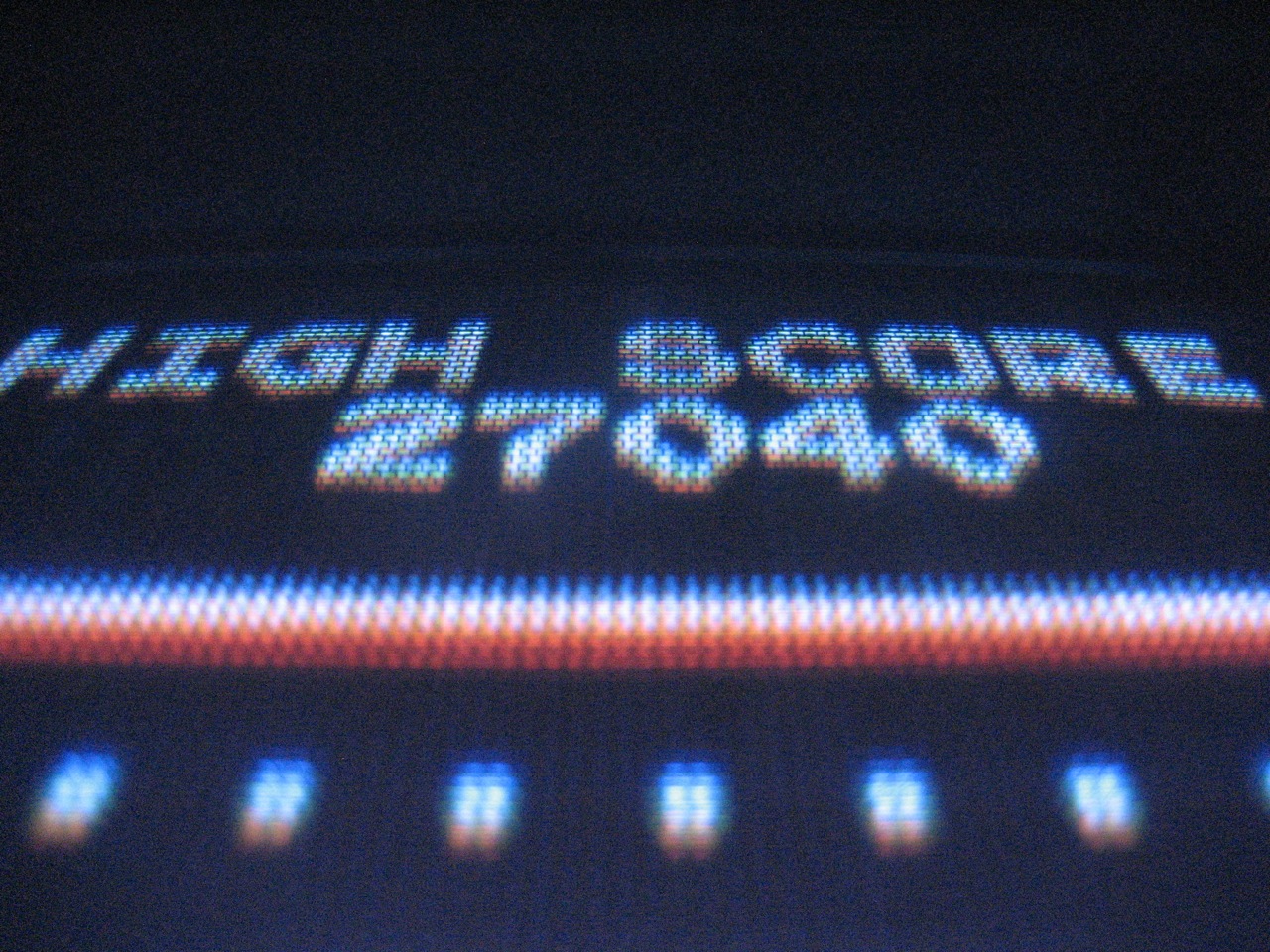In this image, we see a close-up view of a vintage arcade game high score display. The high score of 27,040 is prominently shown in bold, white typography against a solid black background, characteristic of 80s or early 90s arcade games. Below the high score, there is a distinct line consisting of red, white, and blue segments, with smaller rectangular dashes of the same colors extending across the bottom. The old-style pixelated graphics appear grid-like and lack modern detail, enhancing the nostalgic feel. The overall image is black except for the illuminated elements and is somewhat blurry and staticky, suggesting it was captured with an old camera or features low-quality lighting.